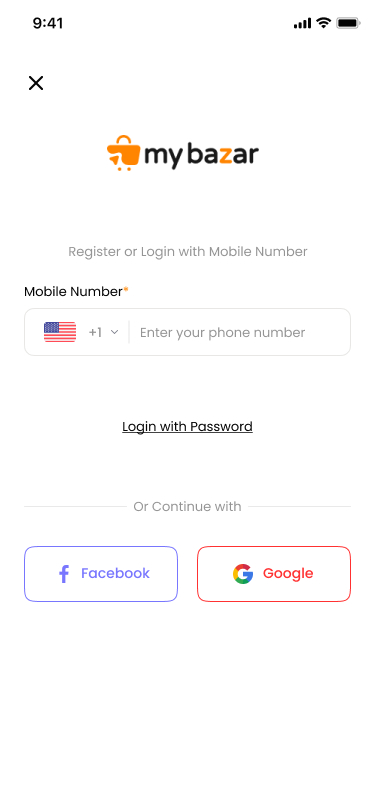The image captures a snapshot of a login page from a cell phone. In the top left corner, the time is displayed as 9:41. In the top right corner, there are icons indicating battery level and Wi-Fi signal strength. At the top center, the logo and name "MyBazaar" are prominently displayed, with the "Z" in "Bazaar" highlighted in orange. Accompanying the name is an icon resembling a suitcase.

The primary focus of the screen is a center-aligned input field designed for entering a phone number, accompanied by a United States flag and a +1 country code. Beneath this input field, there's a link allowing users to log in with a password.

Towards the bottom of the page are two side-by-side buttons for alternative login methods. One button features the Facebook logo, while the other displays the Google logo, both positioned under the text "or continue with." The entire login page is set against a white background, maintaining a clean and minimalist design. This image serves as a clear depiction of the login interface for the MyBazaar application.